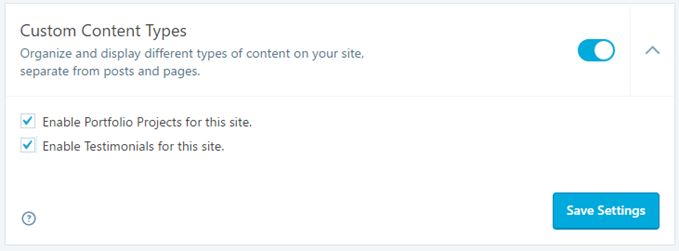The image showcases a user interface snippet from an app or a website with a 3:1 width-to-height ratio. At the top left, the title "Custom Content Types" is prominently displayed in large, black font with the first letter of each word capitalized. Just below, a smaller, blue-gray font text reads, "Organize and display different types of content on your site, separate from posts and pages." To the right of this section, there is a toggle switch in the 'on' position, indicated by the teal-colored background on the left side of the toggle. Adjacent to the toggle, a gray up arrow is positioned.

Below, on the left side, there are two checkboxes, each filled with a blue check mark. The first checkbox is labeled "Enable Portfolio Projects for This Site" in black text, with each of the first three words capitalized. The second checkbox is labeled "Enable Testimonials for This Site," also in black text, with each of the first two words capitalized. At the lower left corner, a black question mark encased in a circle is present, while the lower right corner features a "Save Settings" button in white text against a light blue background.